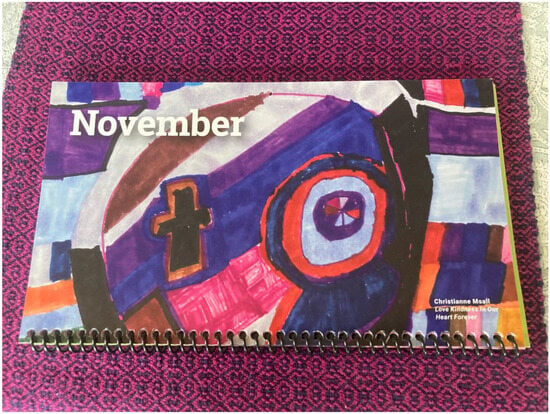The image showcases a spiral-bound lookbook positioned so that the black spiral binding runs horizontally along the bottom edge of the picture. The cover of the lookbook prominently features the word "November" in a serif style font situated in the top left corner. Below this, there is a black cross, and to the right of the cross is a circular pattern with a blue edge, transitioning through orange, gray, and purple towards the center. The center of the circular design contains several small, colorful triangles in shades of red, purple, pink, and brown. The lookbook rests on a magenta fabric that has a diamond pattern composed of both large and small diamonds. The fabric's surface shows a combination of black and purple, enhancing the contrasting geometric patterns and vivid colors on the lookbook's cover.